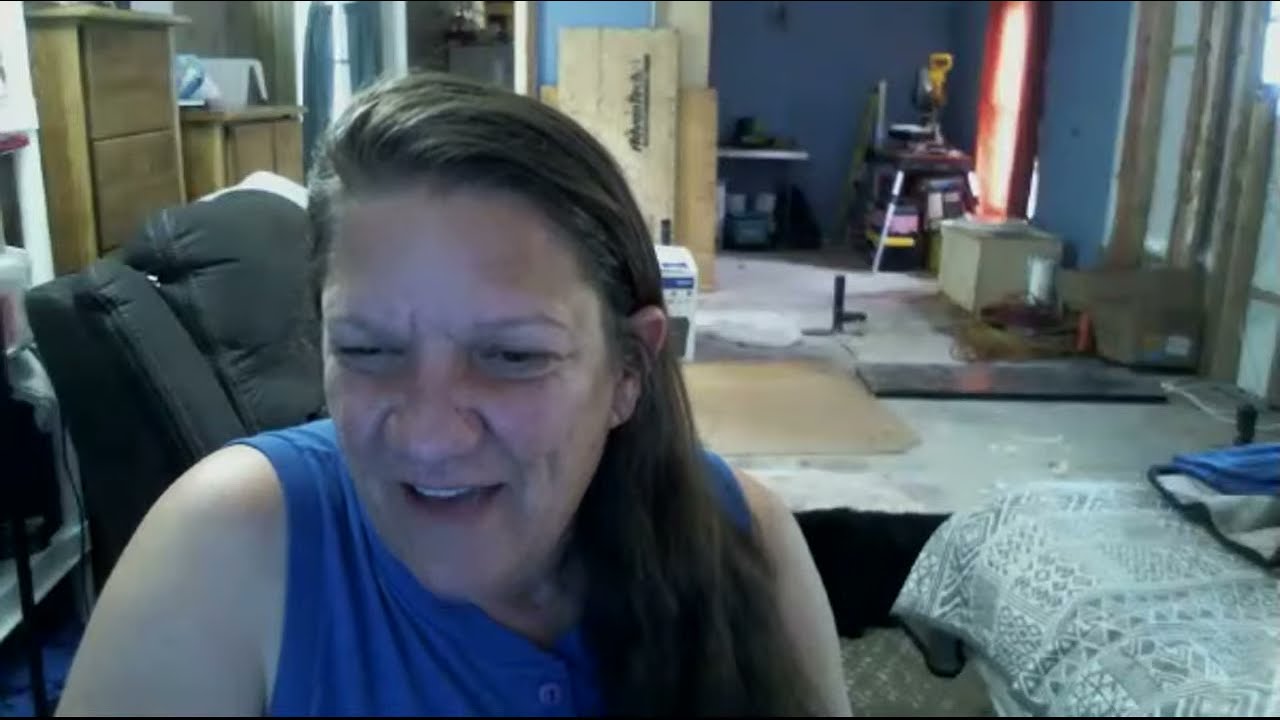The image captures a lower-resolution screenshot of a middle-aged woman engaging in a video blog on YouTube, noticeable by the bluish tint and off white balance of the photograph. The woman, who has long, dark brown hair parted to the side, is wearing a blue sleeveless shirt and appears to be sitting in a black chair. She looks focused and possibly squinting, likely commenting on something on her computer screen. The setting is a room with blue walls and various pieces of furniture, including a table, a couple of wooden chests, and a bed with a white, gray, and teal blanket. Additional details suggest the presence of red curtains over a window behind her, and there are brown cabinets visible in what seems to be an adjacent kitchen. There also appears to be some construction material like plywood on the floor, hinting at possible ongoing renovations. The woman appears engaged and intent, either smiling or talking through the webcam.